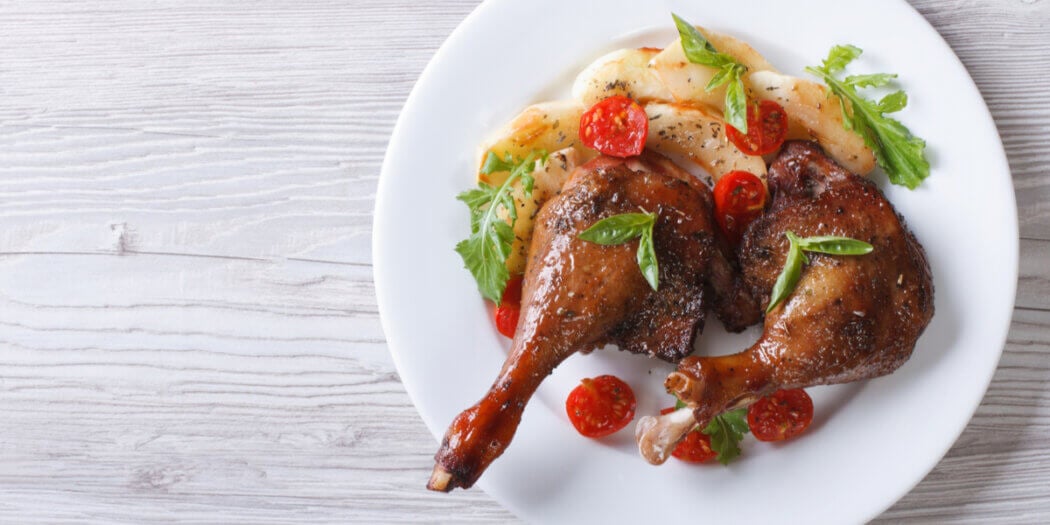The full-color, horizontally rectangular photograph artistically captures a thoughtfully presented meal on a white-painted wooden table, which features a noticeable crack running across its surface. Positioned predominantly on the right side of the image is a white plate holding a delectable serving of braised and browned chicken, specifically the leg and thigh pieces, seasoned with black pepper and possibly other spices. The chicken, with its crispy skin revealing bones at the ends, is surrounded by vibrant, halved cherry tomatoes and a scatter of leafy green garnish. At the top of the plate, there's a portion of white, textured food—potentially potatoes or noodles—adding to the intricate and appealing presentation of this culinary delight.